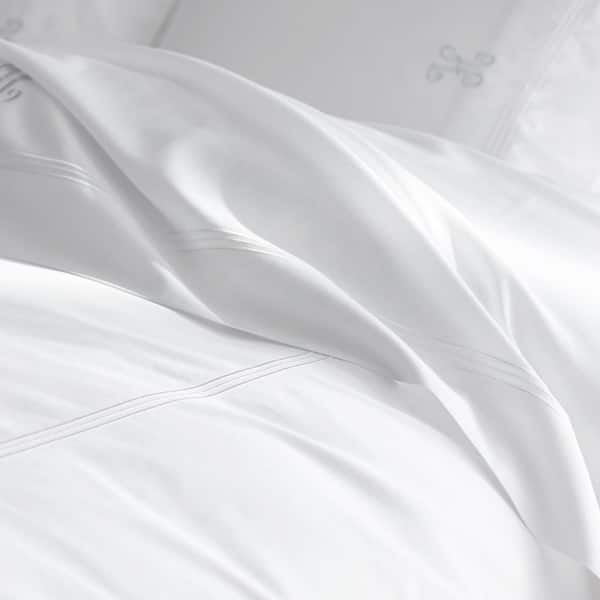This highly detailed, close-up image showcases the pristine bedding of a well-made bed, highlighting the intersection where the crisp white sheets meet the similarly white comforter and pillows. The forefront is dominated by the smooth, high-thread-count sheets that have been immaculately folded over, revealing a glimpse of the flawless surface beneath. Just behind this layer, a white pillow features a graceful, cursive capital "H" on its right side, adjacent to a neat vertical seam, while a partially obscured "H" appears to the left, hidden by a perfectly arranged fold in the sheet. 

The lighting in the photo is bright and professional, enhancing the intricate details and smooth textures of the fabric. This sophisticated setup includes a stitched accent with three vertical lines running horizontally across the folded sheet near the pillows, a design mirrored in the pillow patterns that vaguely form a curving "X," suggesting an abstract branding or decorative element. The cascading folds of the sheets to the right extend towards the bed's edge, adding to the luxurious, inviting presentation of the bedding arrangement.